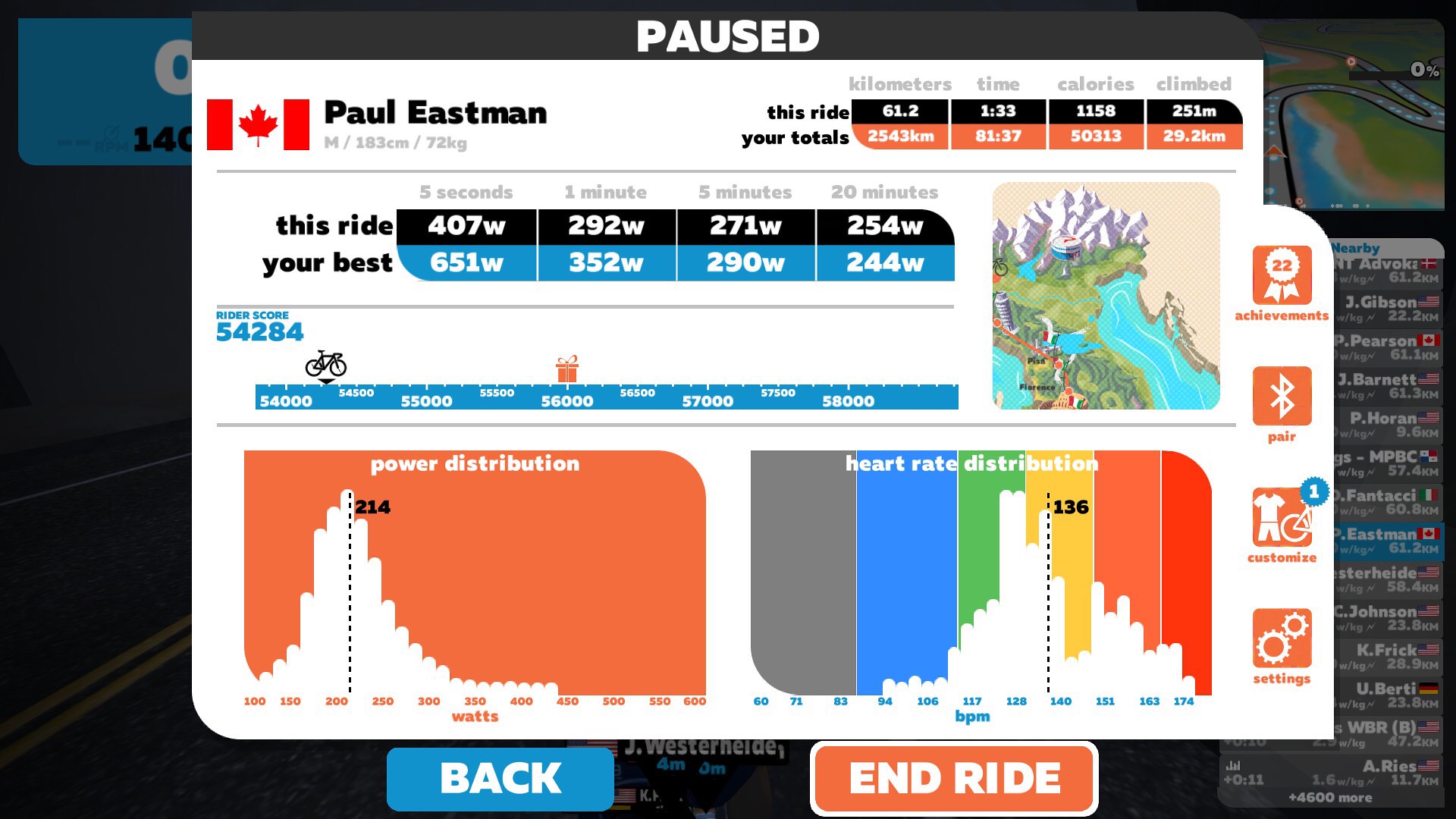This is a detailed display of a workout tracking interface, possibly from a personal computer or connected app monitoring a bike ride. At the top, the status shows "Paused" in large letters. On the top left, there is a Canadian flag icon next to the name "Paul Eastman" along with his details: male, 183 centimeters, 72 kilograms. The screen monitors numerous metrics for the session, labeled as "This Ride" with statistics including kilometers, time, calories, and altitude climbed. Additionally, it compares performances over time intervals of 5 seconds, 1 minute, 5 minutes, and 20 minutes against Paul's personal best records.

Central to the display is a graphical representation of a cyclist and a corresponding ride score. Below that, there are two bar graphs: the left is orange and shows "Power Distribution," while the right illustrates "Heart Rate Distribution." A map in the top right likely depicts the route taken during the ride. Towards the bottom of the screen, there are interactive options such as "Back" and "End Ride". Other buttons on the right side include "Achievements," a Bluetooth pairing icon, "Customize," and "Settings." The comprehensive interface is intricately designed to provide a detailed overview of Paul's cycling performance and progress.